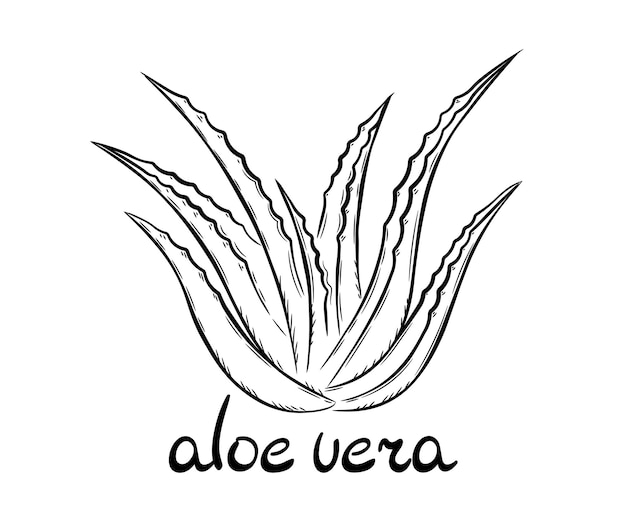The image is a simple and minimalistic black-and-white drawing of an Aloe Vera plant. The background is pure white, emphasizing the stark outline of the plant. Below the image, in black cursive-like text, the words "Aloe Vera" are written, providing clear identification. The Aloe Vera plant is depicted with long, pointed leaves that have jagged edges on one side, resembling but differing from lettuce due to the spiky nature. The leaves are primarily concentrated at the center, with two large leaves flanking a close-knit pair in the middle, another two extending outwards, and a single leaf pointing towards the center. The overall layout of the leaves creates a fan-like arrangement, with sharp, black tips that are a characteristic feature. This simplistic illustration, almost clip-art-like, captures the essential elements of the Aloe Vera plant, making it easily recognizable.